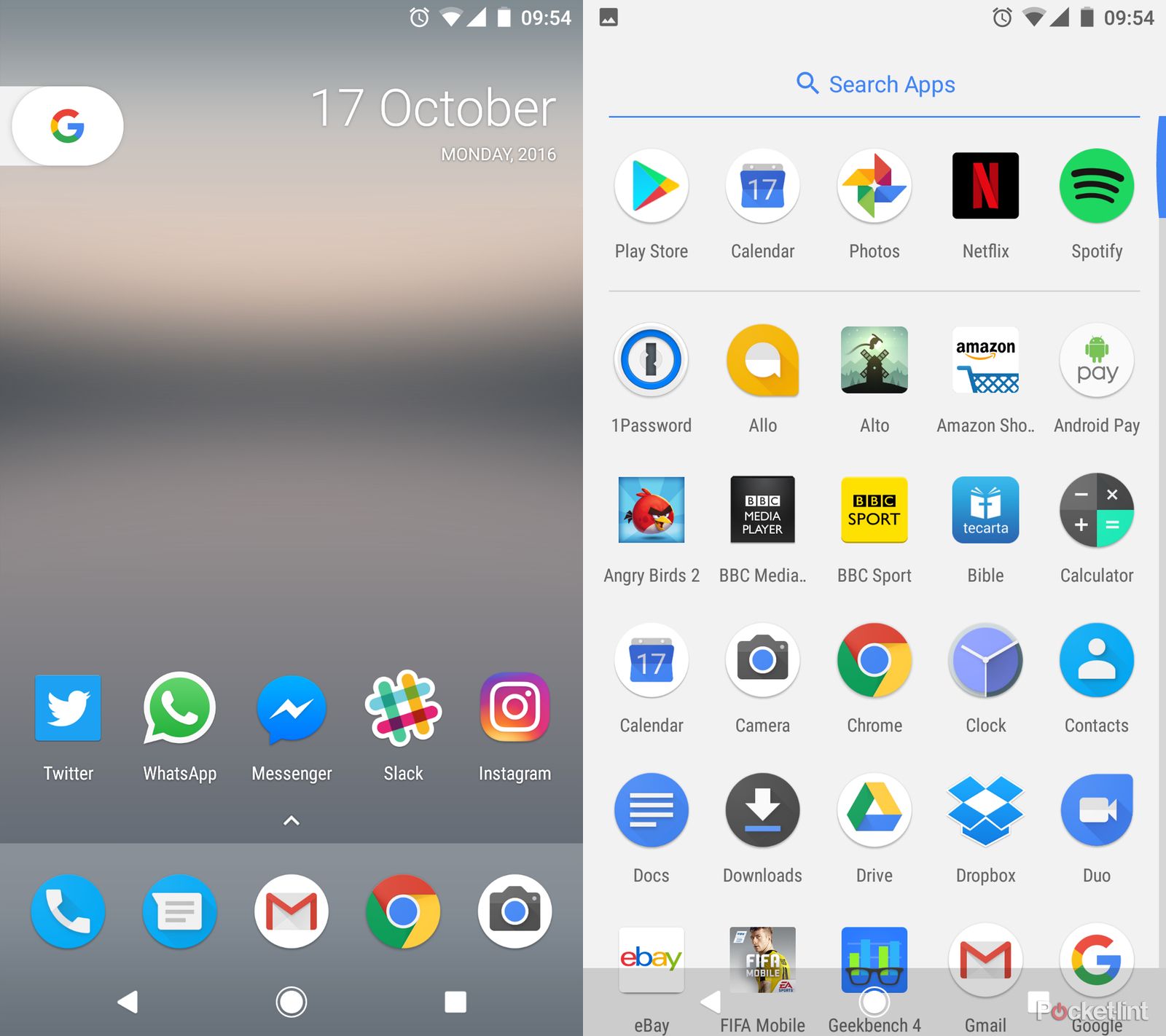This image is a detailed screenshot of a mobile device's homepage and app menu, likely taken on October 17th, 2016, a Monday. On the left side of the screenshot, phone options are visible along with a small Google icon at the top. Central to the display are easily recognizable app icons including Twitter, symbolized by a bird within a box, WhatsApp with its familiar phone icon, Messenger, Slack, and Instagram. Additional app icons shown below include the phone's messaging app, Google, Chrome browser, and a camera application.

Beside the main screen, an extended view reveals a secondary screenshot, potentially indicating either a larger device like an iPad or two side-by-side screenshots from a single phone. This expanded view showcases a vast array of neatly organized apps against a pale gray background, featuring applications from the Play Store, Calendar, and others. Noteworthy mentions include Password Manager, Angry Birds, Chrome (appearing again), Amazon Shopping, Dropbox, Contacts, Geekbench 4, and various gaming apps. BBC Sports and BBC Media Player are also part of this comprehensive app collection. The overall impression is a meticulously arranged overview of the user's downloaded apps.